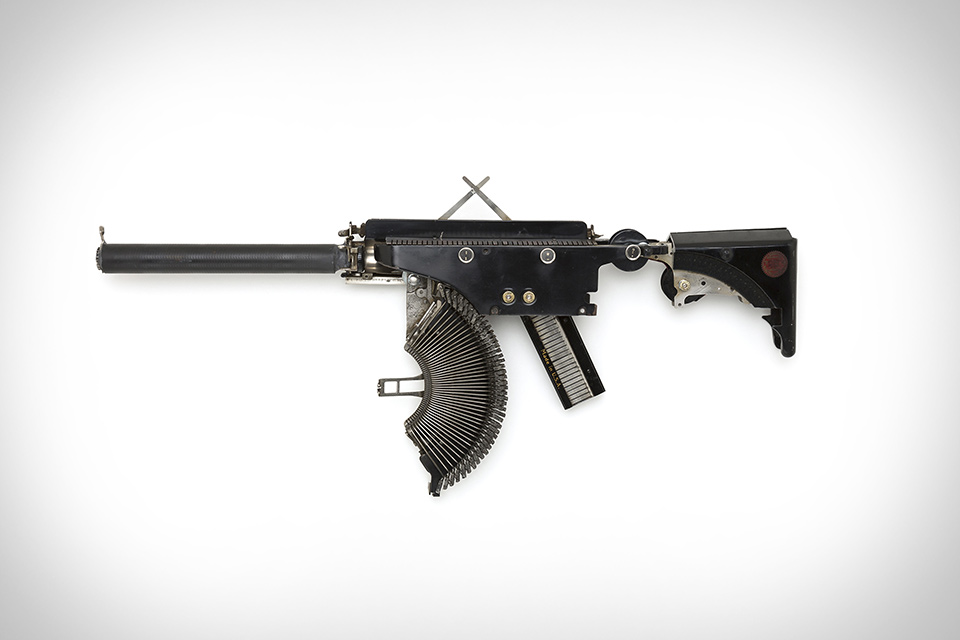The image depicts an intriguing contraption, primarily black in color, showcasing a blend of various textures and components. The base of the device features a semi-circular design reminiscent of a half-fan, while the top portion is adorned with pointed, spiky elements. These spikes have ridged, textured edges that add to the intricate design. 

On the right side, a section of the contraption is made from sleek, slightly shiny black leather. Towards the bottom, a rectangular component protrudes at a diagonal angle. This piece is divided into three sections: the top and bottom sections are black, matching the main body, whereas the center is a striking silver. 

The leftmost edge of the contraption terminates in a cylindrical, tube-like structure, entirely black, adding to the complex and multifaceted appearance of the device.